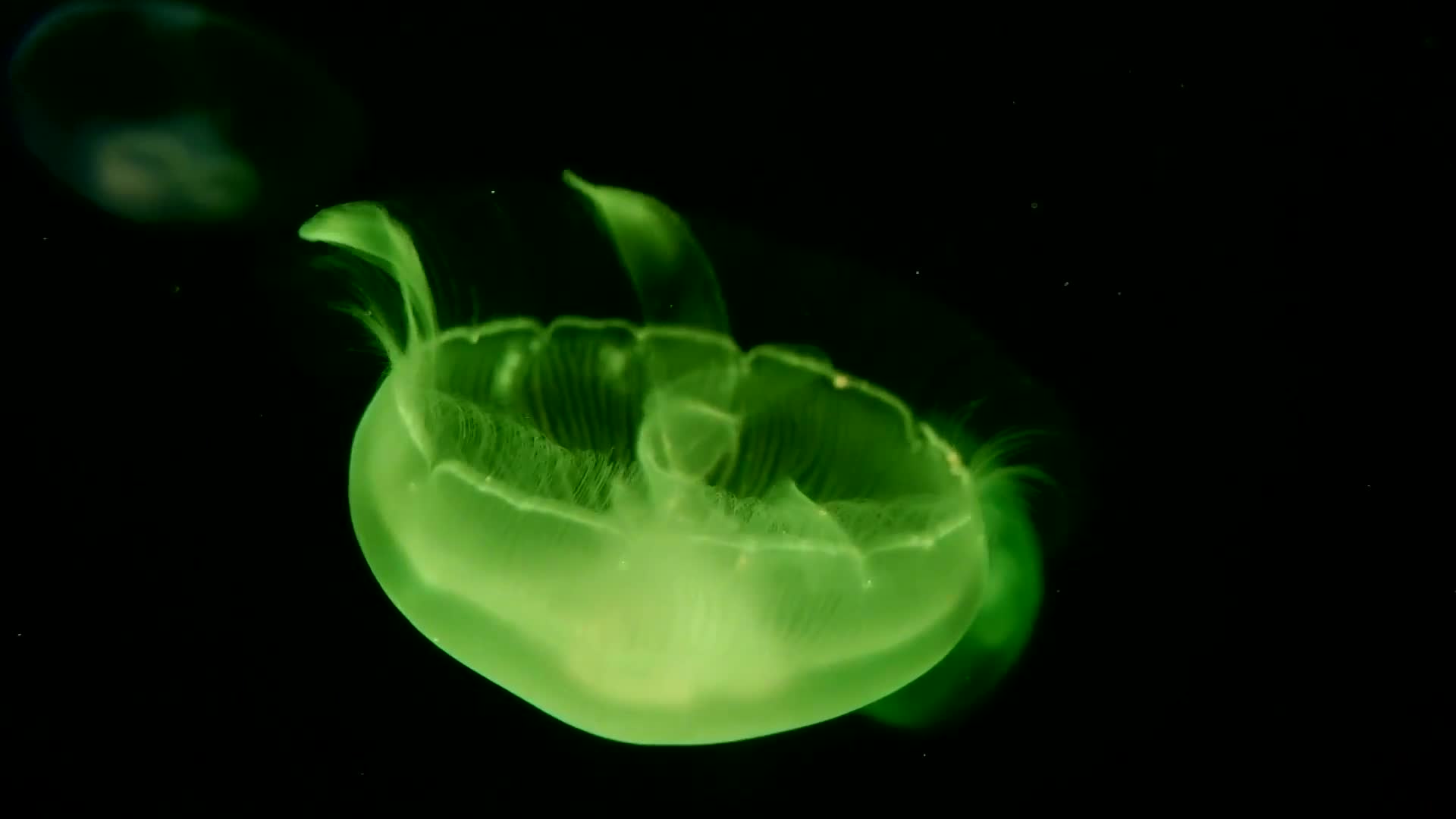This captivating bioluminescent image showcases an ethereal jellyfish bathed in a vibrant light green glow against a completely black background. The jellyfish appears upside-down, resembling a bowl or an upside-down mushroom, with its bottom visible on top. Its semi-transparent body reveals a brighter central area, emitting a mystical luminescence. Two flat tendrils extend from the bottom of the bowl-shaped creature. The lip of the jellyfish is irregular and features cutouts, adding to its otherworldly appearance. In the faint upper left-hand corner, a blurry silhouette hints at the presence of another jellyfish, further enhancing the depth and mystery of the scene. The overall black backdrop contrasts sharply with the jellyfish, making its delicate features and intricate details stand out exquisitely.